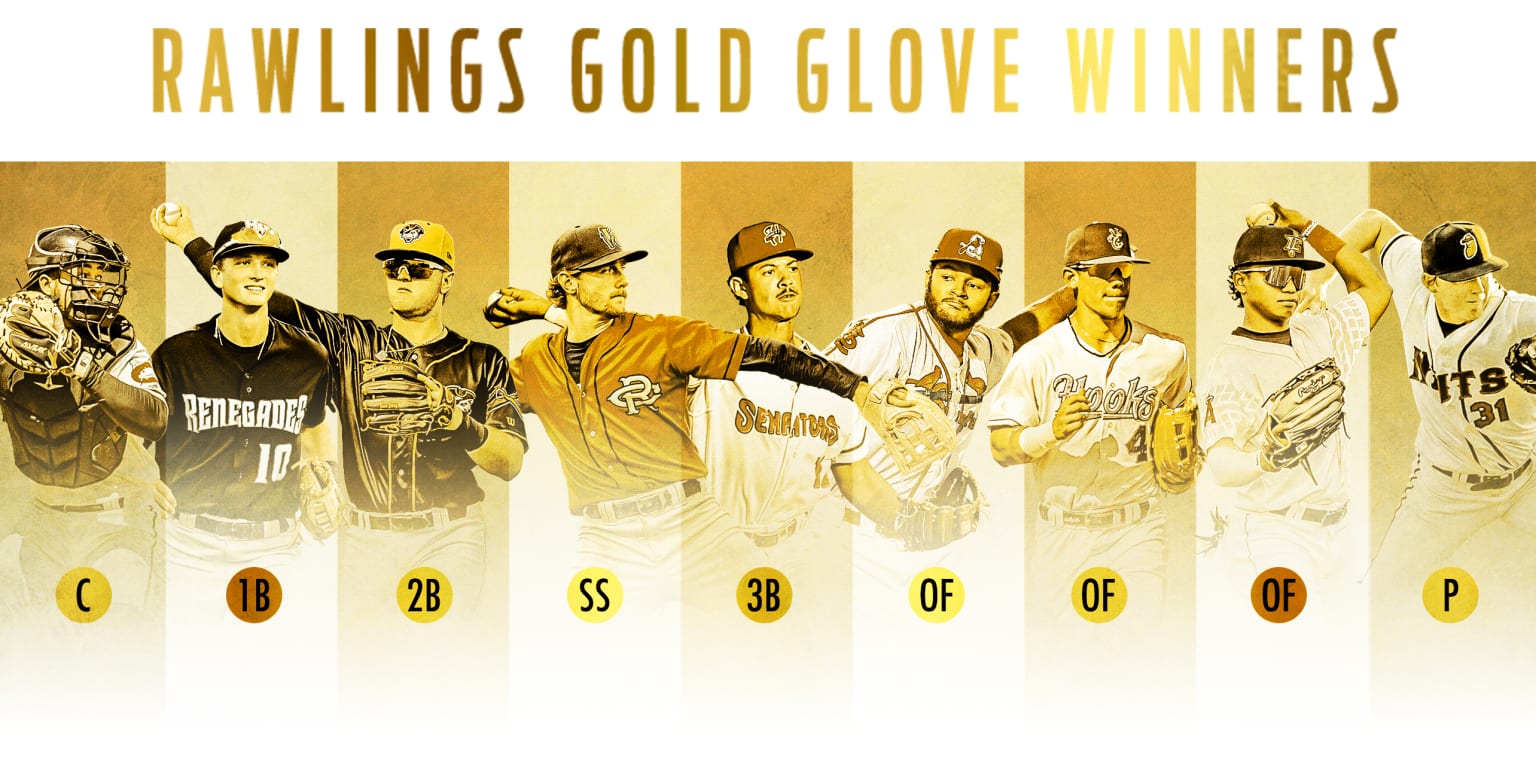The image is a detailed stylized poster showcasing the Rawlings Gold Glove winners. At the top of the poster, written in a gradient of gold and dark yellow text, is "Rawlings Gold Glove Winners." Below this heading, an array of baseball players is displayed, each in the midst of an action shot. From left to right, the players represent the following positions: catcher (C), first baseman (1B), second baseman (2B), shortstop (SS), third baseman (3B), three outfielders (OF), and a pitcher (P). Each player is distinguished by a position abbreviation encircled beneath their image. The players are dressed in various uniforms, indicating different teams: the predominant colors include white, black, red, and orange jerseys. The catcher stands out with a helmet, while the other players sport baseball caps, and some also wear sunglasses. Behind each player, the poster features either a gold or white stripe, contributing to the overall aesthetic. The background fades into white at the bottom, adding a clean finish to the composition.